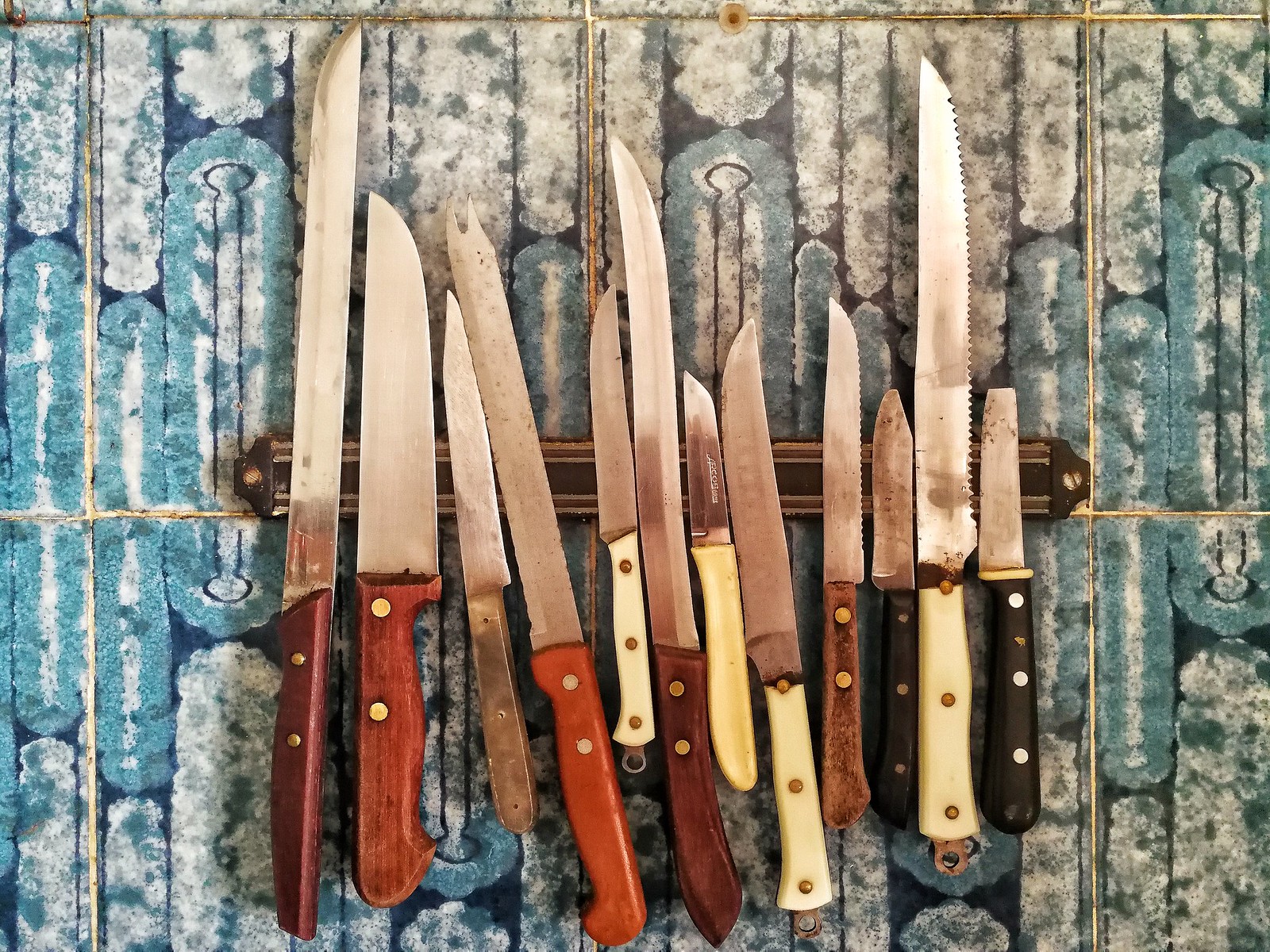This image depicts a collection of 12 assorted kitchen knives displayed on a horizontally-mounted magnetic strip on a wall. The magnetic strip is affixed to a tile background with an eclectic blue and white pattern featuring elongated oval shapes. The tiles and the grout appear dingy and are marked with signs of wear and dirt, suggesting a well-used kitchen environment. The knives vary in type, including steak knives, paring knives, serrated blades, bread knives, and cheese knives. They are assorted in size and length, with handles in different materials and colors—such as black, white, natural wood, and yellowish plastic. Some knives show signs of age and disrepair, with rust spots and a disheveled appearance, indicating they are quite old and have seen extensive use. One knife on the far right even has a broken tip. The overall photo is brightly lit, though the colors are not very vibrant, likely due to high contrast and an ample amount of natural light streaming in from a nearby window.